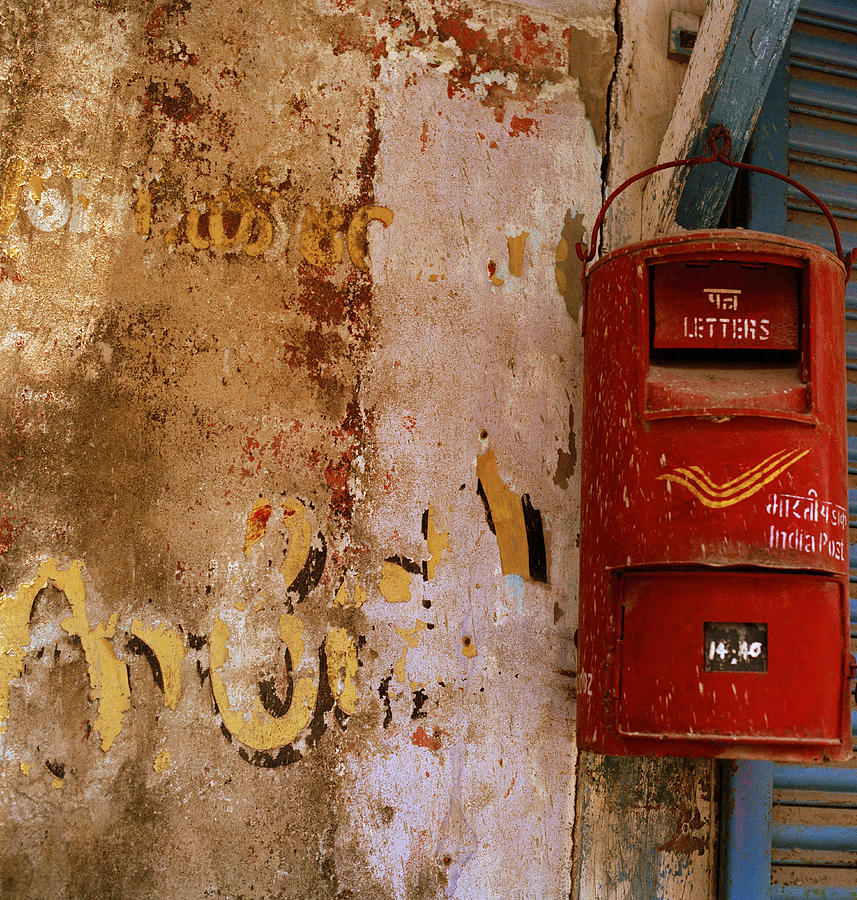Close-up image of a weathered concrete wall reveals remnants of various colored murals, graffiti, and posters, which have been repeatedly stripped away and repainted. Dominating the right side, a red, elongated mailbox, labeled "LETTERS" in white English letters and additional text in a foreign language, hangs from a blue beam. This mailbox, appearing dusty and well-used, features two flaps for mail delivery and collection—one for putting mail in and one at the bottom that opens to the left for retrieving mail. Below this, a blue ladder is visible in the bottom right corner. The wall itself displays shades of white, yellow, and red, with evidence of natural light illuminating the scene, possibly indicating a city environment that's been seasoned with time.